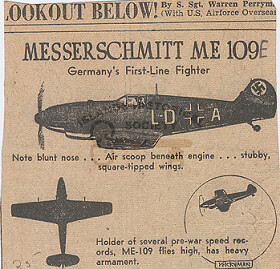The image captures an aged, yellowing snippet from an old newspaper or promotional flyer, featuring a detailed account of the World War II Messerschmitt Me-109E, Germany's first-line fighter. The headline, "LOOK OUT BELOW!", accompanied by a credit to SSGT Warren Perry, U.S. Air Force Overseas, draws attention at the top. The central focus is on a black-and-white illustration showing multiple views of the aircraft—including side, bottom, and angled perspectives. Notable features such as the blunt nose, air scoop beneath the engine, and stubby square-tipped wings are highlighted. The plane, marked with a swastika on its tail and annotated with "LDA", is noted as a holder of several pre-war speed records and known for flying high with heavy armament. Additional text provides historical context and technical specifications.